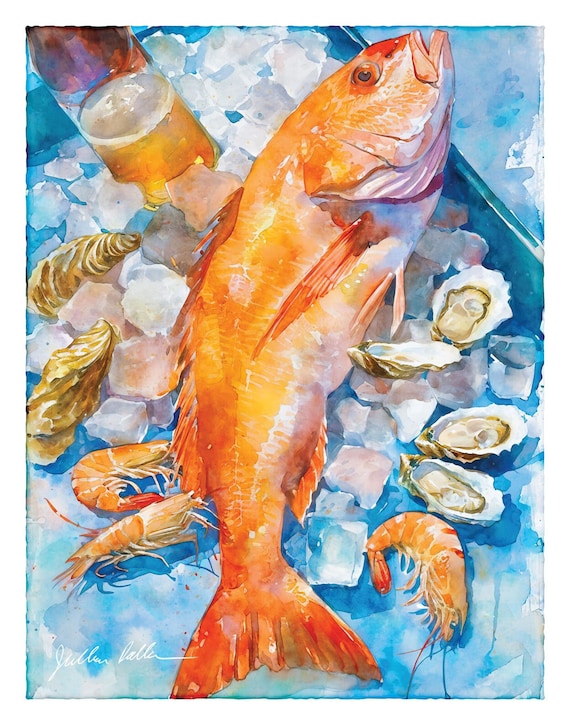The image is a semi-realistic painting with watercolor-like effects, primarily focusing on a large, golden-orange fish lying on its side atop a bed of chunked ice. The fish, with its head pointing towards the top and its tail towards the bottom, features vibrant hues of orange, yellow, and red, with orange fins and eyes. It's positioned on a blue material, possibly a cooler or plate, surrounded by both open and closed mussel shells in white and brown colors. Scattered around the fish's tail are several unpeeled orange shrimp. Towards the top left, there is a transparent bottle or glass containing a yellow liquid, likely beer or champagne. The background is an abstract mix of blues and whites with swirling patterns. In the bottom left corner, there is a white cursive signature, possibly reading "Jillian" or something similar.